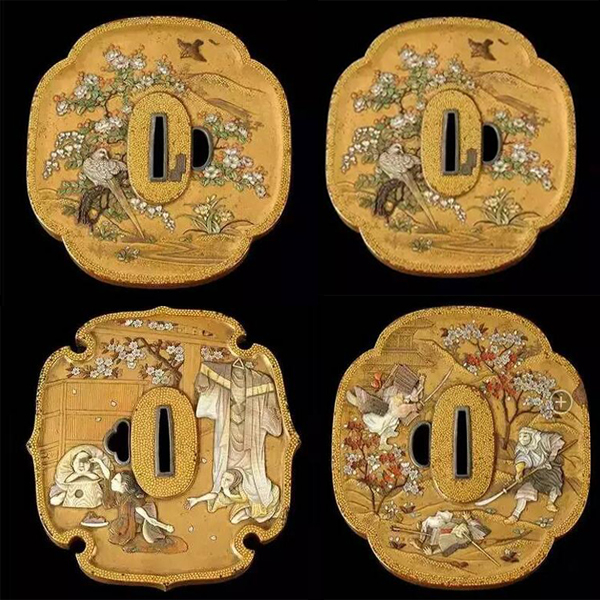The image depicts four ornate, gold-colored objects set against a black background. Each object is positioned in one of the four corners of the image and shares a similar shape: round with a slight indentation resembling a four-leaf clover in each corner. 

The top two objects feature intricate depictions of birds perched on trees adorned with white flowers. The branches are detailed in shades of black and brown, with tan accents adding to the realism.

In the bottom left corner, the object presents a domestic scene: a person with brown hair on their knees under a garment that resembles a kimono hanging on a hanger, while another individual, clad in a darker long garment, reaches towards an adjacent object.

The bottom right features a scene with additional red flowers among the white ones on the trees. This scene involves a more elaborate interior or possibly an outdoor setting with people; one interpretation suggests a woman tending to a man, while another sees it as figures in a field.

Each of these objects contains rectangular holes at their centers, reminiscent of keyholes or apertures. To the side of each central opening, there's another decorative aperture, either a half-circle or a cloud-edged semi-circle, adding to their ornate design. These could potentially be coin-operated slots or keyholes, though their exact function remains ambiguous. Each element combines to suggest an artifact with culturally rich, possibly Asian-inspired, artistic elements.